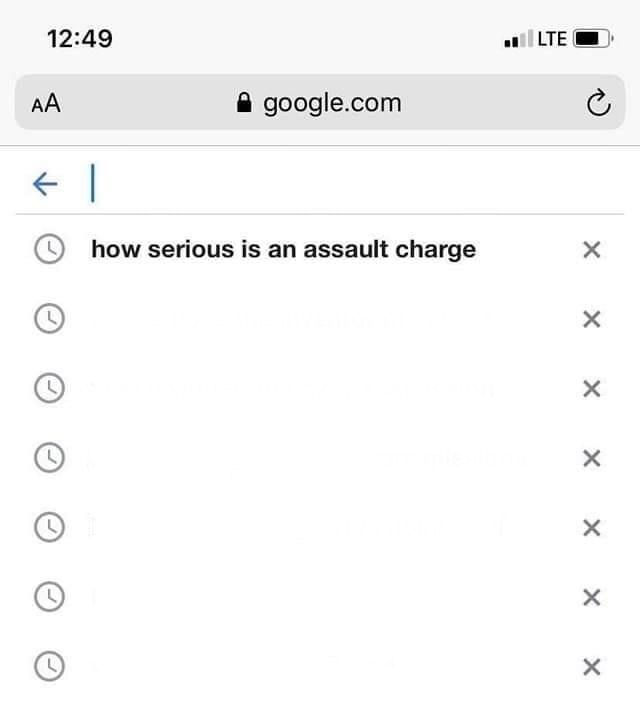Screenshot of a Google Search on a Mobile Phone

The image shows a crucial moment captured at 12:49 PM, as indicated by the clock at the top. The phone is connected to LTE with two out of four bars of signal strength, and the battery is approximately 70% charged. The central focus of the screenshot is a Google search query.

At the top is the URL bar displaying "google.com" secured with a lock icon, signifying a secure connection. Adjacent to the URL bar, on the right, is a small "A" and a larger "A" icon, likely representing text size settings, followed by a circular arrow icon for page refresh.

Beneath the URL bar is a vertical list of search results, which appears incomplete and unusual. There are seven horizontal lines, each marked on the left with a clock icon and on the right with an "X" for closing the result. However, only the first line contains text, stating "how serious is an assault charge" without a question mark. The rest of the lines are blank, displaying no additional text or links.

This anomaly in the search results is peculiar and might suggest an error or a mocked-up interface, as the person notes their extensive experience with Google searches but never encountering such a format. The minimal and incomplete display of search results raises questions about its authenticity or functionality.